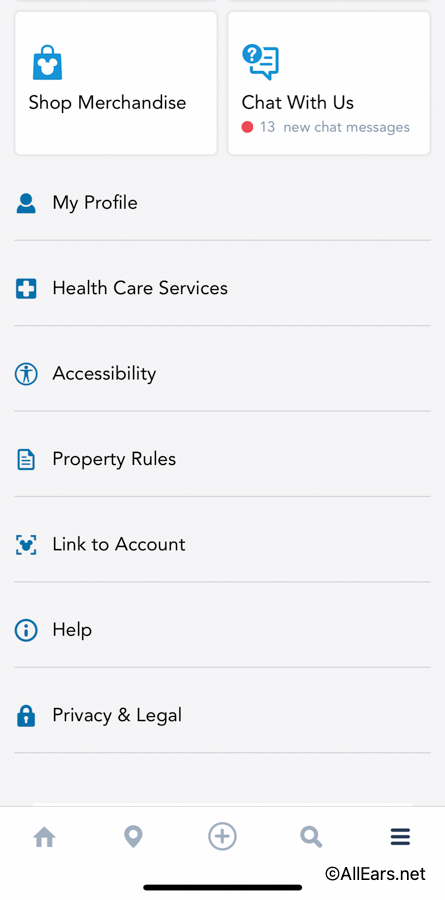This image is a screenshot featuring a section of a website, as indicated by the copyright notice "copyrightallears.net" at the very bottom. At the top of the screenshot are two prominent white squares containing black text and blue icons. The first square is labeled "Shop Merchandise" and features a teal shopping bag icon with a Mickey Mouse head inside. The second square is titled "Chat With Us" and displays a teal chat bubble with a question mark in the top corner. This chat section indicates there are 13 new chat messages.

Below these two squares is a navigational menu comprised of various options. Each option is accompanied by a thin gray line and a respective icon. The options and their corresponding icons are as follows:
- "My Profile" with a person icon
- "Healthcare Services" with a medical band-aid icon in blue
- "Accessibility" with a human silhouette inside a circle
- "Property Rules" with a paper icon
- "Link to Account" with a Mickey Mouse head inside a square
- "Help" with an eye icon inside a circle
- "Privacy and Legal" with a lock icon

This structured layout allows users to easily navigate through different sections dedicated to personal profile management, healthcare information, accessibility, property rules, account linking, assistance, and privacy and legal information.